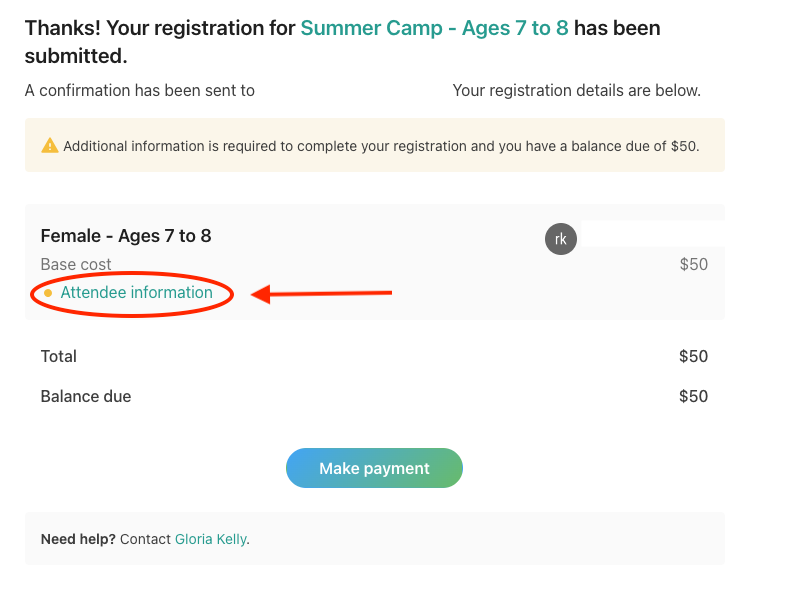This image is a detailed screenshot from a webpage displaying a registration confirmation. The background at the top is white, paired with a dark gray font that reads, "Thanks!" followed by "Your registration for" in black font. The phrase "summer camp, ages seven to eight" is prominently written in green font, and then it continues in black font with "has been submitted."

Below this main message, in smaller, gray font, is a note, "A confirmation has been sent to," but the email address is not visible in the screenshot. On the right side of the image, there is a note saying, "Your registration details are below."

A light pink rectangle spans the width of the image, containing a gold triangle warning symbol with a white exclamation mark, signifying an alert. This section informs the user, "Additional information is required to complete your registration," and mentions "You have a balance due of $50."

Beneath this alert, on the left side against a white background, the information is laid out: "Female - ages seven to eight" is in bold font, followed by "base cost" in gray. The "attendee information" is highlighted with a red oval and pointed to by a red arrow. Below this, it says "total" in gray, and directly on the right side is the balance of "$50" in green font. The specific balance due area shows "$50" again, indicating the remaining amount owed.

At the bottom-center of the screenshot is a rectangular button with rounded corners, split into blue and green halves, labeled "Make payment" in white text. On the left side, gray font prompts, "Need help? Contact Gloria Kelly," where "Gloria Kelly" is a blue hyperlink, suggesting it can be clicked to reach assistance.

This detailed layout suggests the payment is pending, and additional actions are needed to complete the summer camp registration for ages seven to eight.